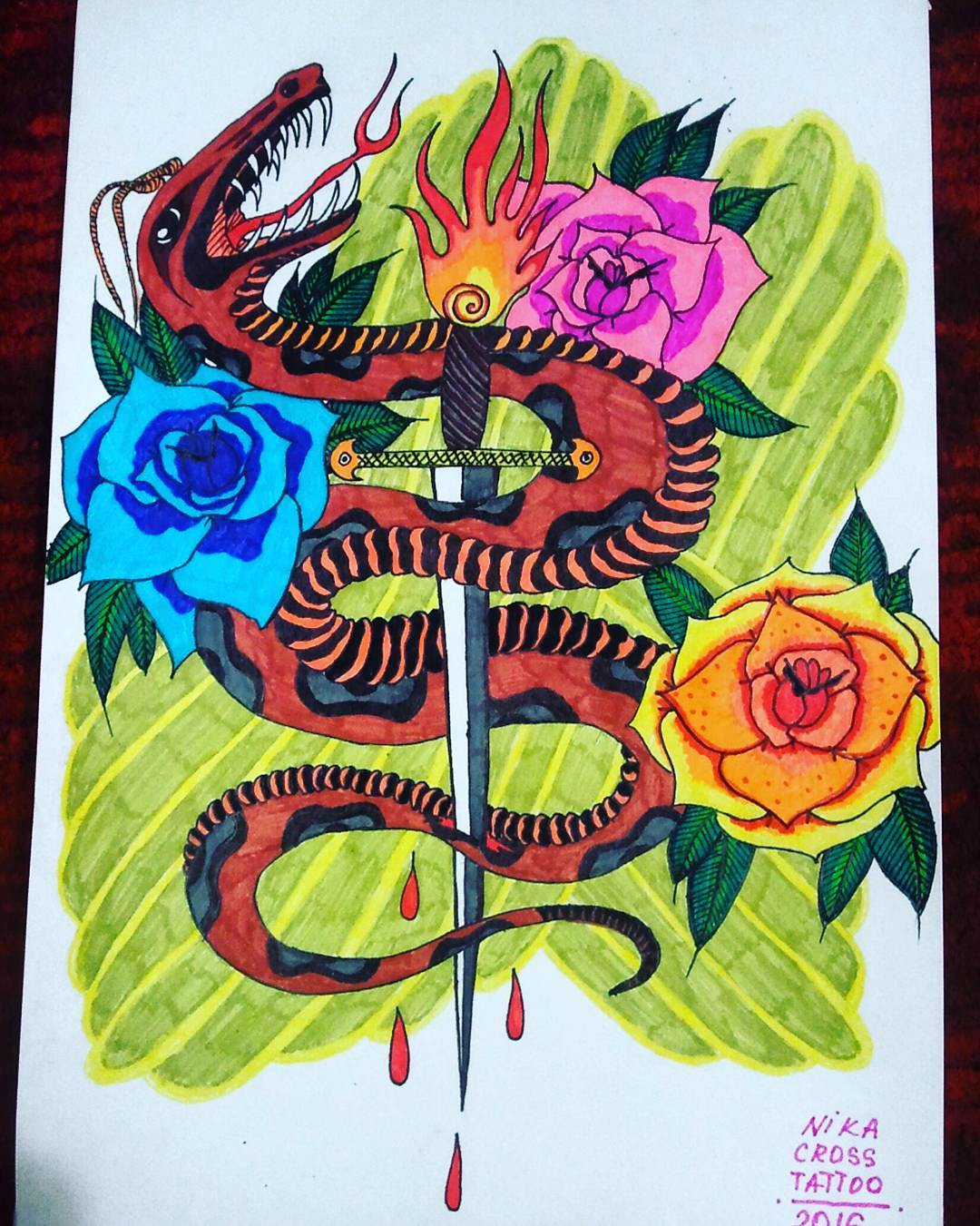The image is a vibrant, hand-drawn sketch on white artist's paper, set against a dark brown background. The main focal point is a sword with a black handle and a silver-blue blade, which is depicted pointing downward. This sword is intricately wrapped by a serpent-like creature that resembles a lizard or dragon. The creature is primarily red with black spots, and it features an alternating red and black pattern on its underbelly. Its exaggerated mouth is open, revealing numerous teeth and a forked tongue. The blade of the sword appears to be dripping red blood where it pierces the creature's back.

Surrounding the central motif are three vividly colored flowers: a blue rose, a pink rose, and an orange-yellow rose. The background is filled with an arrangement of green shapes and leafy patterns, along with yellow stripes, enhancing the overall complexity and beauty of the design. In the lower right-hand corner, the text "Nika Cross Tattoo 2016" is inscribed in pink, suggesting that this might be a design intended for a tattoo.